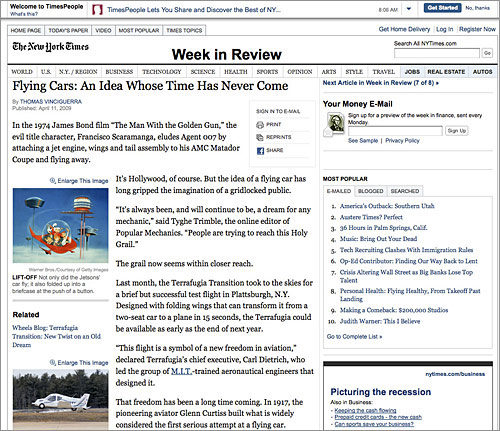"Welcome to Timed People, a platform that lets you share and discover the best of New York. Featured in New York Times Week in Review, the age-old fascination with flying cars is revisited. The 1974 James Bond film, 'The Man with the Golden Gun,' showcased the villain Francisco Scaramanga escaping in a modified AMC Matador Coupe, equipped with a jet engine and wings. This Hollywood fantasy has long captivated a gridlocked public's imagination. 'It's always been and will continue to be a dream for any mechanic,' says Taggy Trimble, online editor of Popular Mechanics. The dream now seems close to reality. Last month, the Terrafugia Transition conducted a successful test flight in Plattsburgh, NY. This innovative vehicle features folding wings, allowing it to transform from a two-seat car into a plane in just 15 seconds."